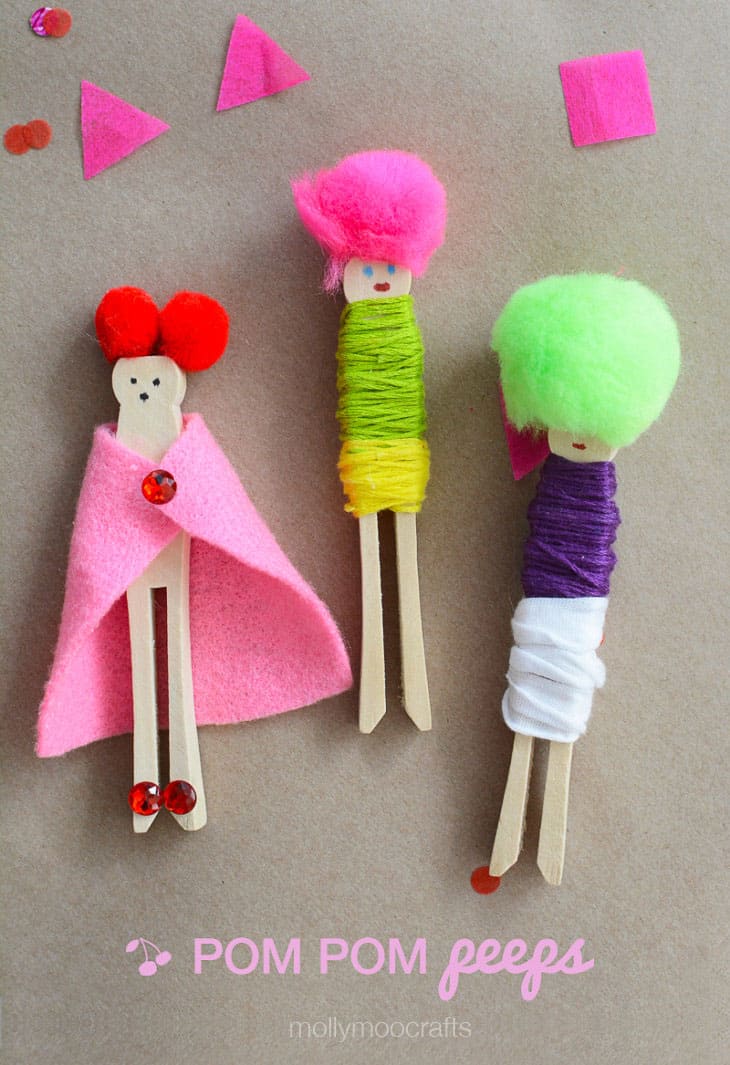The image showcases a delightful arrangement of three handcrafted doll clips, ideal for craft enthusiasts. The dolls are made from light wooden clothespins, each featuring unique, brightly colored pom-poms atop their heads, representing hair. These figurines have tiny faces drawn on the wooden surface and are adorned with various fabrics and yarn wrapped around them, mimicking clothing. The clip on the left flaunts a set of red, round gemstones and wears a pink felt cape. Another clip is dressed in bright green and yellow yarn, creating the look of a green shirt and yellow shorts. The third clip includes accents of purple and white. The dolls are set against a light gray background that resembles felt, adding texture to the presentation. Above the dolls, tiny red felt circles and pink geometric shapes, including triangles and a square, create additional visual interest. At the bottom of the image, in bold pink letters, the text reads "POM-POM PEEPS," with "Molly Moo Crafts" written underneath in white cursive. A charming pink cherry icon accompanies the text on the left side.